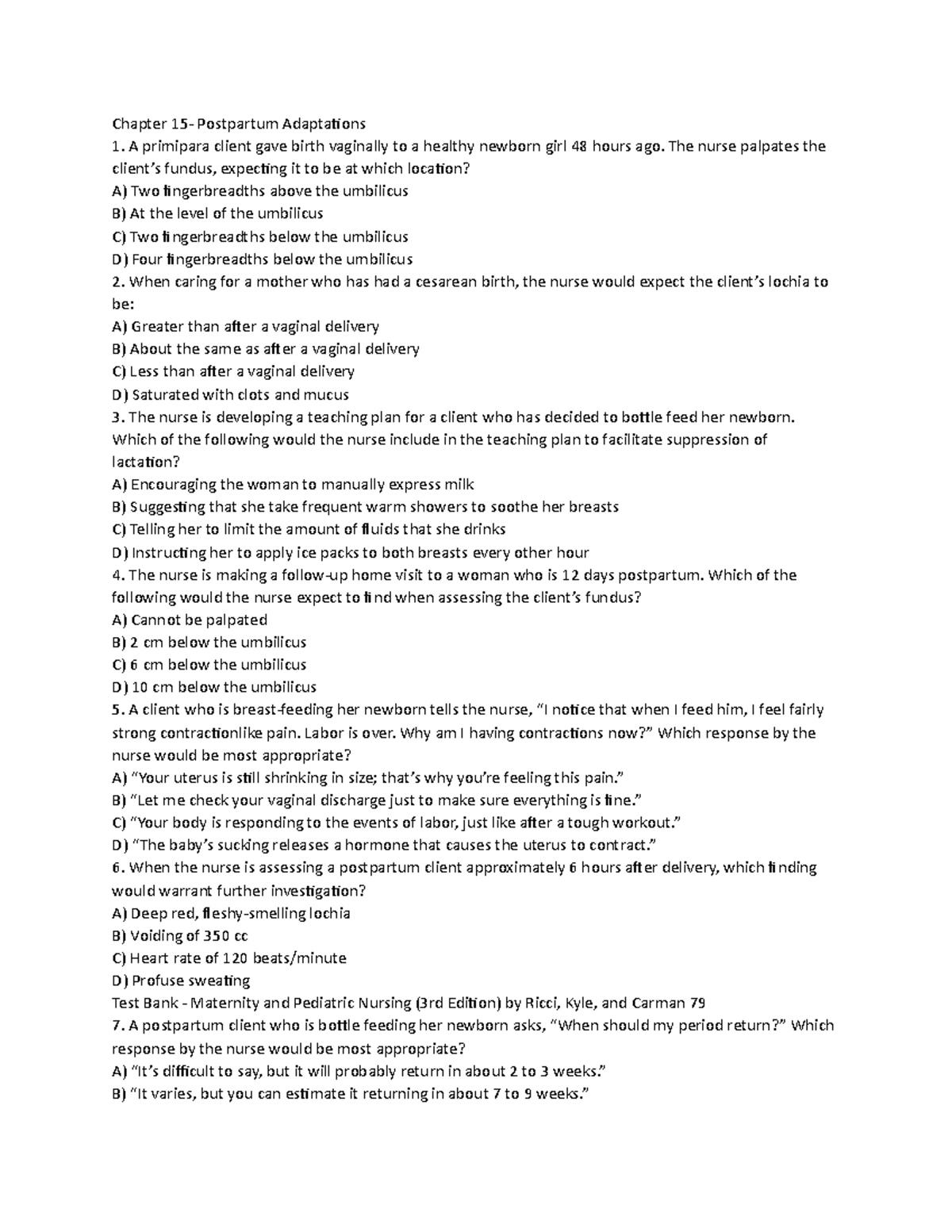On a plain white background, the image depicts a text-heavy page titled "Chapter 50: Postpartum Adaptation." The page features a series of numbered multiple-choice questions, organized sequentially from 1 to 7. Each question presents a statement or scenario followed by four answer choices labeled A, B, C, and D, except for the last question, which only offers options A and B. 

For instance, one of the questions discusses care for a mother who has undergone a specific type of birth, prompting the nurse to anticipate certain client responses. Another detailed segment addresses the development of a teaching plan for a client who has chosen to bottle-feed her newborn. The plan includes recommendations such as limiting fluid intake to facilitate a particular aspect of the lactation process.

This image exemplifies a detailed examination or study guide focused on postpartum nursing care and patient education.